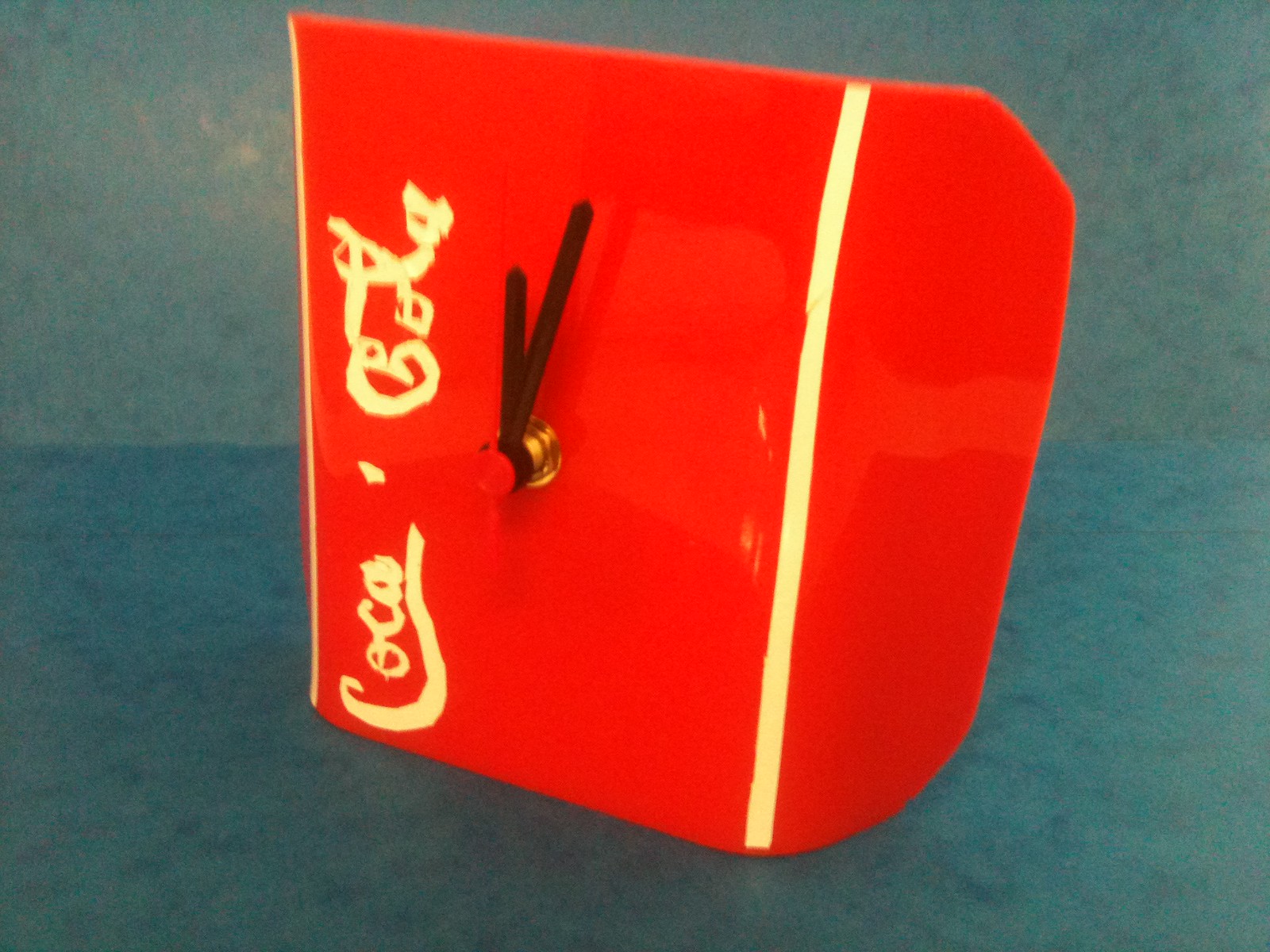This close-up photograph showcases a unique, red clock set against a blue-gray, mottled background. The clock features a distinctive square design with the upper right-hand corner cut off diagonally. A thin yellow strip lines the left edge of the clock, adjacent to a section with what appears to be either Chinese or Arabic script. At the center of the clock is a yellow-gold circle, from which two black hands, an hour and a minute hand, extend. Notably, the clock lacks a second hand and numerical markers. On the right side of the clock, there is a prominent, thick yellow line extending vertically from the top to the bottom, but it does not reach the edge of the photograph.